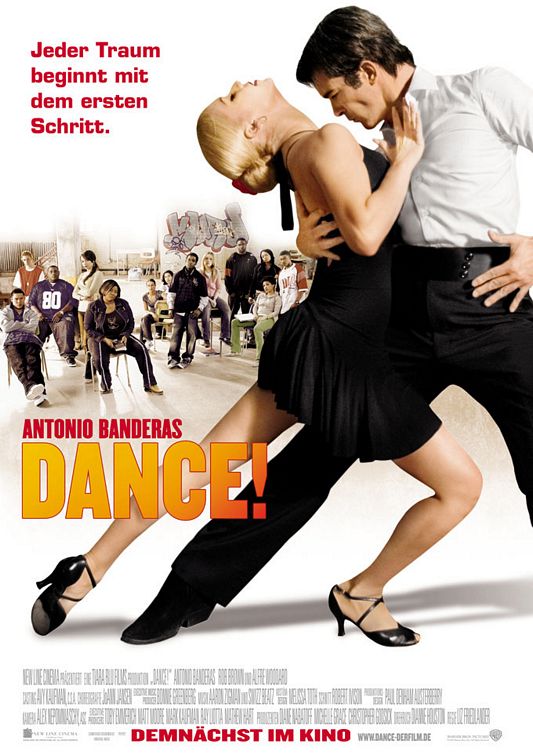The poster showcases Antonio Banderas in a dramatic dance pose with a woman, likely promoting a foreign-language movie about dancing, as the title, written in bold orange with an exclamation mark, is not in English. He is dressed sharply in a white long-sleeve button-down shirt, black pants, a black belt with three buttons, and black dress shoes. His dance partner, a blonde woman, is clad in a short, black dress that laces around the neck and black heeled dance shoes. They are depicted in a passionate stance with the woman arched backwards and their legs extended. The backdrop features an audience of seated or standing onlookers, possibly students in a graffiti-adorned room, who appear disinterested and disengaged. This setting suggests the scene might be from a dance competition or a dance instruction session.